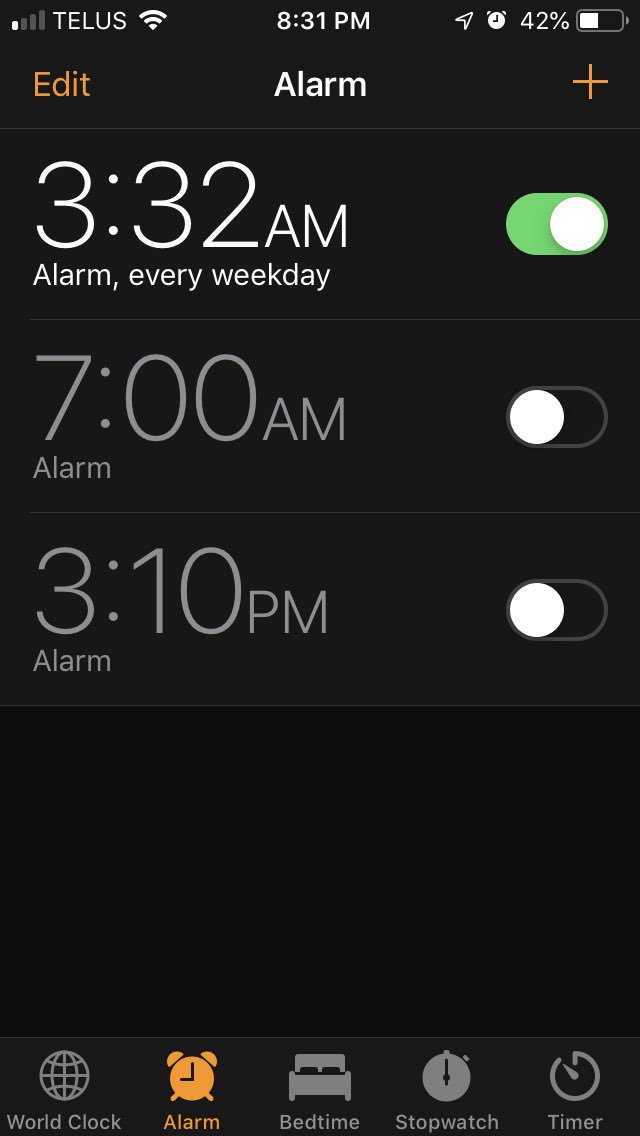The image showcases a smartphone interface in portrait mode, featuring a dark theme with white text on a black background. 

In the top-left corner, white icons for reception and Wi-Fi strength are displayed, alongside the text "TELL US." Centrally situated is the time, "8:31 PM." On the top-right, there is a right-pointing arrow symbol, a white alarm clock icon, the percentage "42%," and a half-full battery icon.

Directly below, the word "Alarm" appears in white text, with a yellow "Edit" button on the left and a yellow plus symbol on the right. The first listed alarm reads "3:32 AM Alarm Every Weekday" in white text with a green, switched-on button to the right. Following it, the "7:00 AM Alarm" is written in gray, accompanied by an off button. Below that, "3:10 PM Alarm" is displayed, also in gray with an off button.

At the bottom of the screen are navigation options depicted with corresponding icons. These include a globe for "World Clock," a clock for "Alarm," a bed for "Bedtime," a stopwatch for "Stopwatch," and a dial for "Timer."